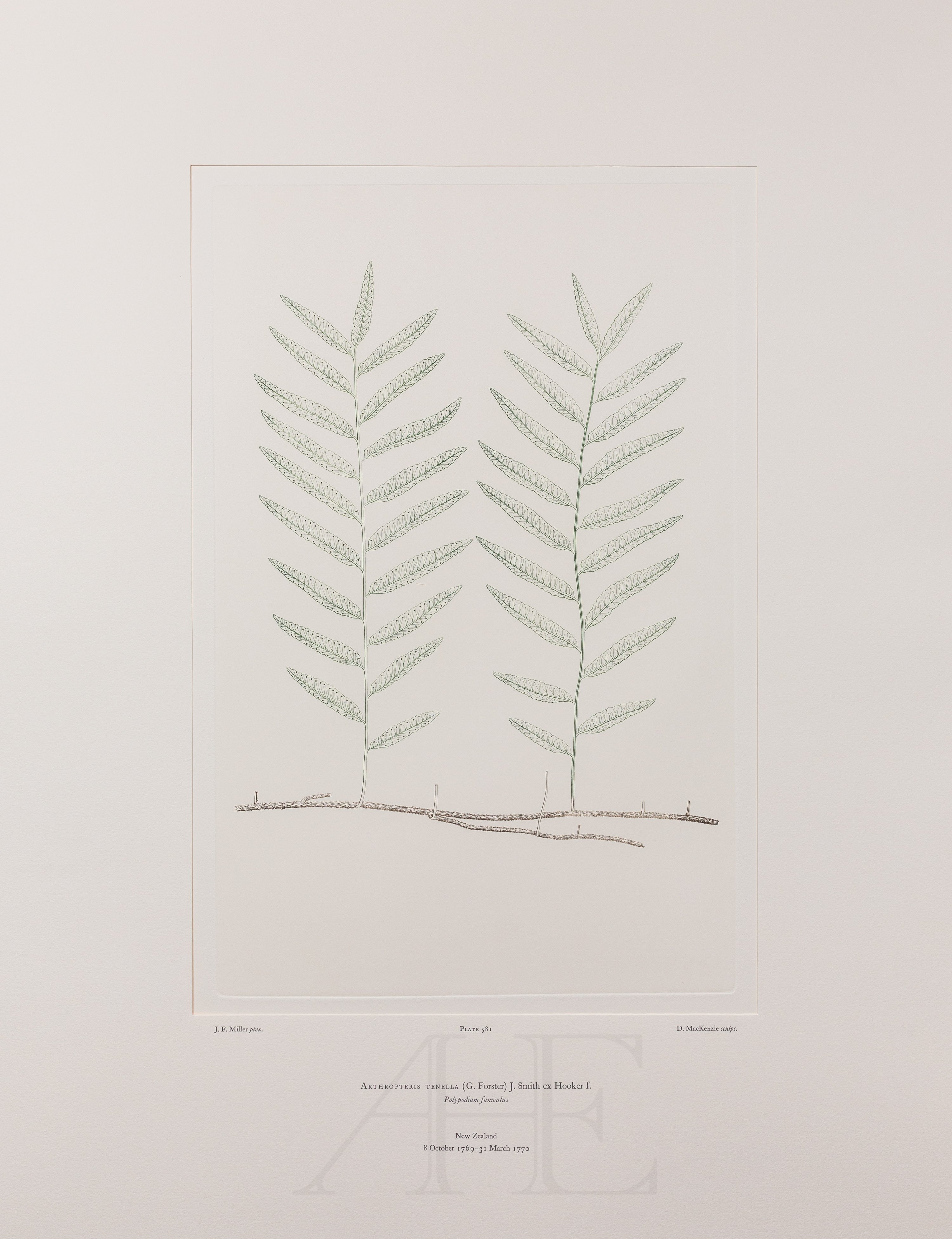This detailed artwork features a meticulously illustrated plant mounted on a wide white mat with a beige background. The sketch depicts two identical, sharply shaped green leaves with a lacy pattern, standing vertically from a horizontal, thin brown branch that appears to have been drawn with pencils. The botanical illustration is highly detailed, giving the leaves a realistic and textured appearance. Accompanying the leaves on the bottom of the paper are several inscriptions, including the artist's name, J.F. Miller, the plate number 381, and D. McKenzie. Additionally, the artwork lists the plant's species, Arthropteris tenella, alongside its scientific classification. The text also notes the location as New Zealand and dates ranging from October 8, 1769, to March 31, 1770, suggesting it records historical botanical details.